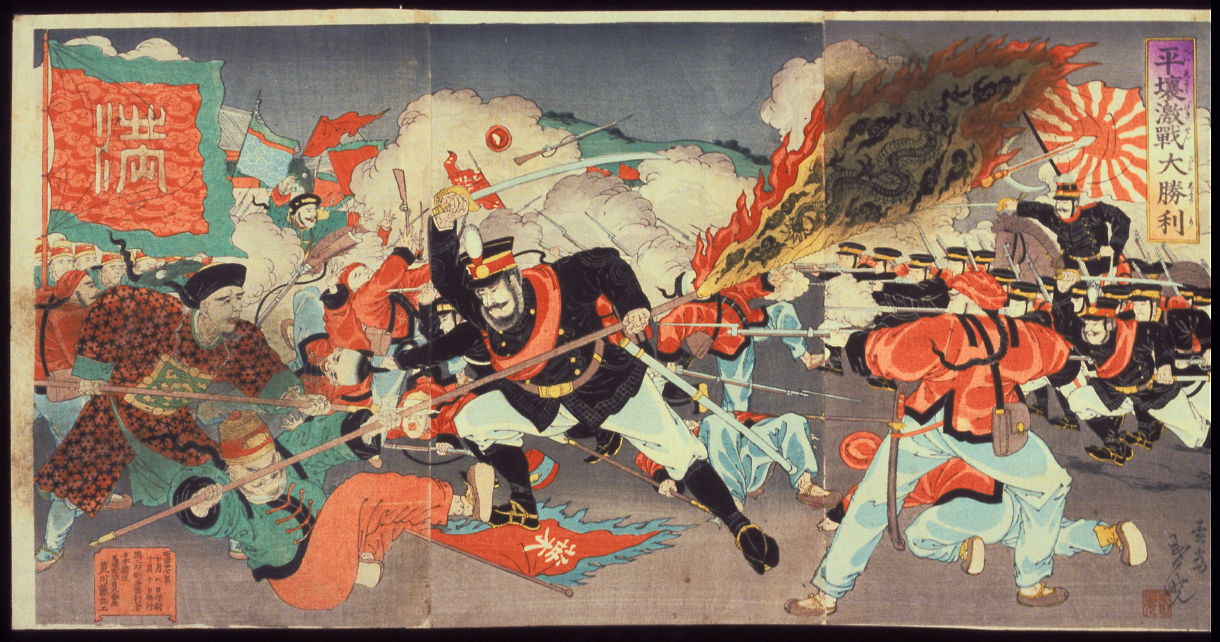This image is an old, Japanese wartime artwork that exhibits significant wear and tear, including creases, as if it had been folded or reassembled from three pieces. The scene is a chaotic battle, showcasing an army of men clashing fiercely. Central to the composition is a prominent figure donned in a black jacket, white pants, and black boots, wielding a long staff from which a yellow flag flutters. This flag bears black artwork and is dramatically encircled by flames. The central figure, also brandishing a sword above his head, appears to be in a struggle for the flag against multiple adversaries. These opponents, situated predominantly on the right side, are equipped with rifles affixed with bayonets and wear contrasted green and reddish uniforms. On the left, his allies, similarly attired in black jackets and white pants, are seen rushing into combat amidst dense clouds of smoke. The background is awash with turmoil, with burning flags and unreadable foreign text adding to the historical and tragic atmosphere of the artwork.